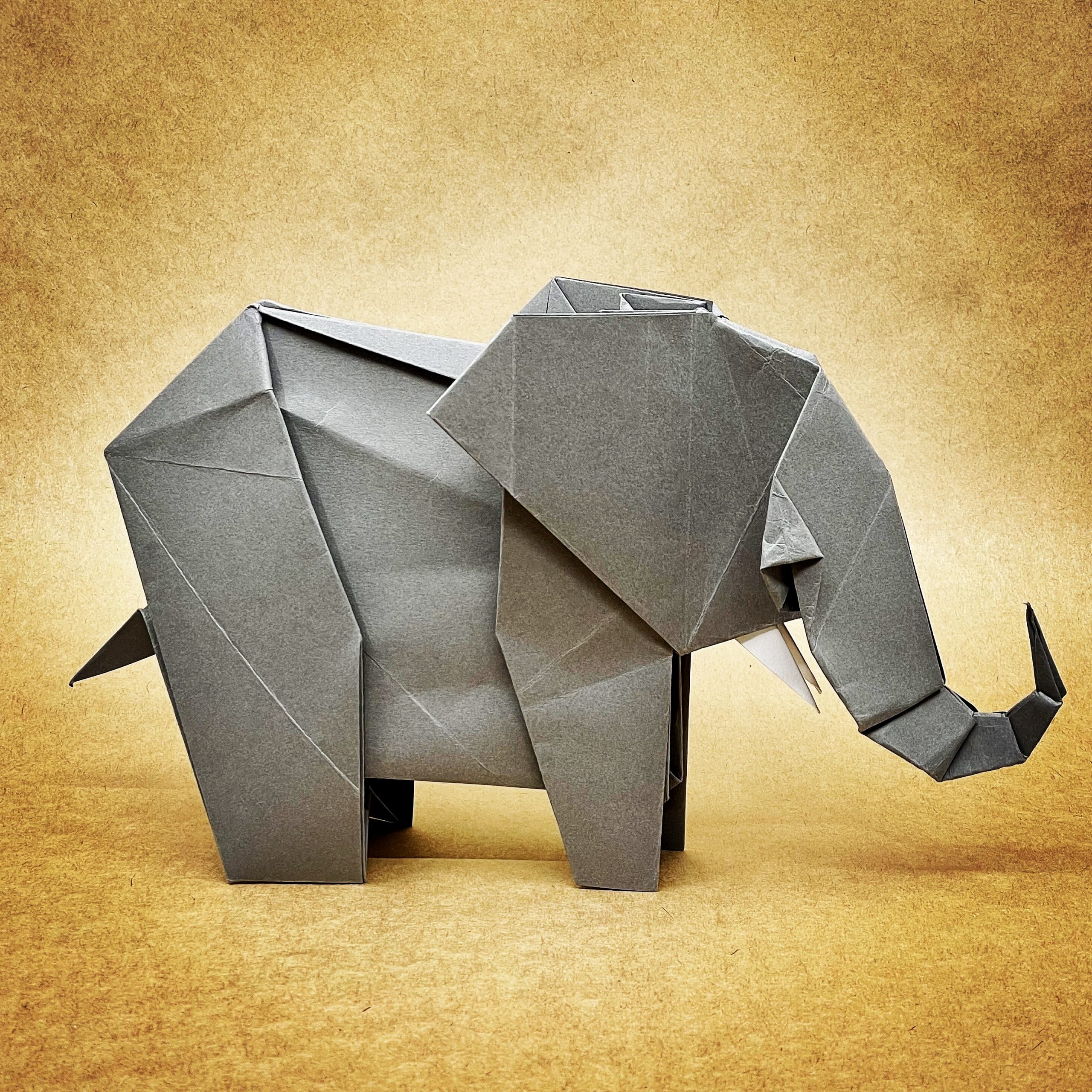This digital artwork features a paper mache origami elephant set against a rich, multi-toned brown background. The background gradates from pale shades near the center to darker browns at the corners, creating a visually engaging frame for the central figure. The origami elephant, crafted from folded gray and dark gray paper, occupies the center of the image. Detailed creases and lines accentuate its folded-paper texture, reinforcing the impression of meticulous craftsmanship. The elephant is oriented so that its back is on the left and its head on the right, with a long trunk that curves downward and then swoops back up in a shape reminiscent of the letter "J." Subtle white paper is used to construct its tusks, which peek out from under its head. A short, pointed tail extends from its left rear. The artwork captures the intricate details of the elephant, making the gray paper stand out vividly against the gradient brown backdrop.